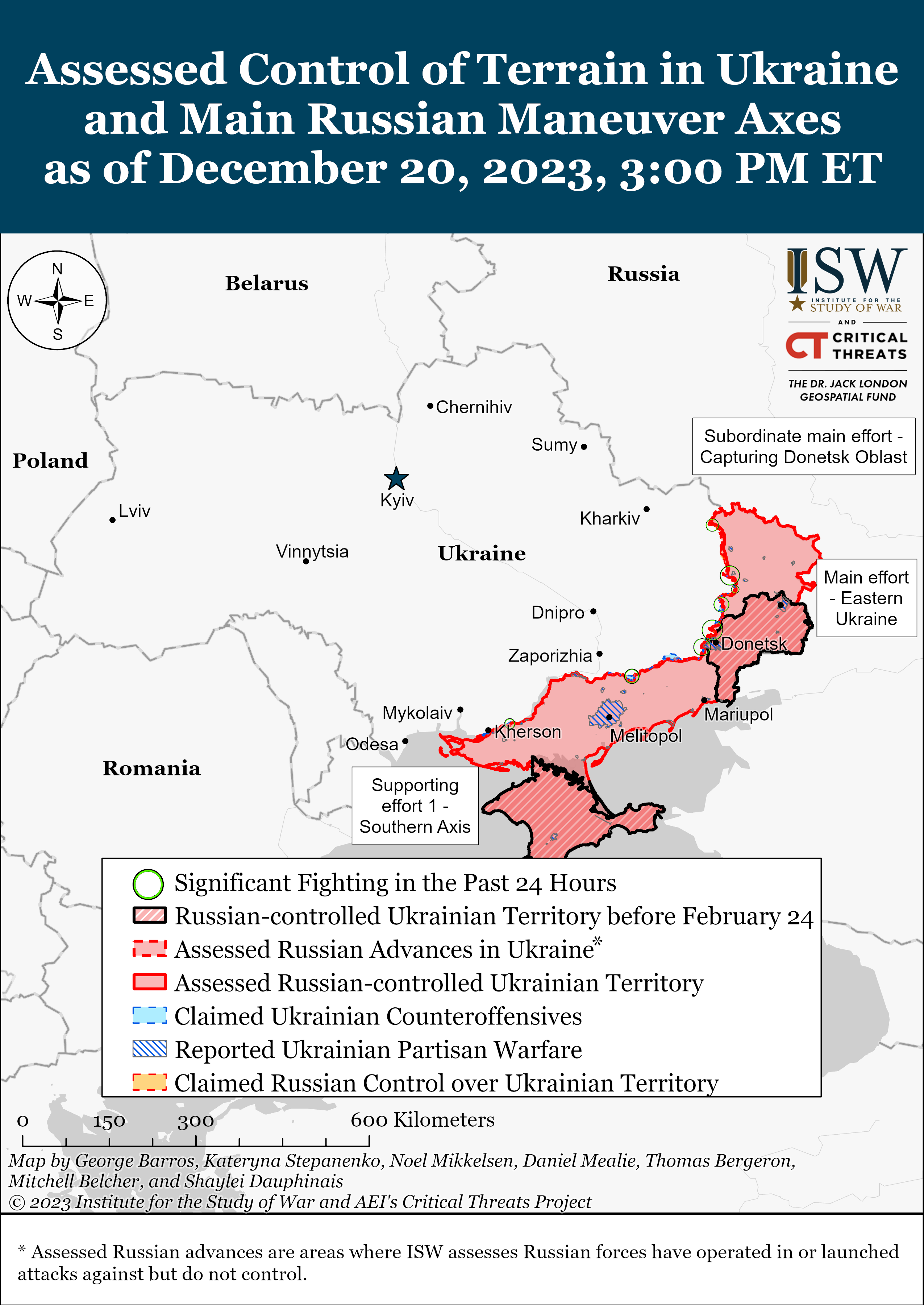A detailed map titled "Assess Control of Terrain in Ukraine and Main Russian Maneuver Axes as of December 20th, 2023, 3 p.m. EST" is bordered by a blue banner with white text. The map primarily features Ukraine and its surrounding countries—Russia, Belarus, Poland, Romania—with areas highlighted in red, pink, and various other colors indicating different levels and types of control and conflict. Key cities such as Kharkiv, Dnipro, Zaporizhzhia, Donetsk, Mariupol, Melitopol, and Kherson are marked.

The map's visual elements include gray dashed country borders, pale pink shaded areas, and red bordered regions indicating Russian advances. Specific symbols denote different aspects: green-circled areas represent significant fighting in the past 24 hours; black rectangles with diagonal red and white lines mark Russian-controlled Ukrainian territory before February 24th. Light blue areas with dashed blue borders indicate claimed Ukrainian counteroffensives, while gray bordered sections represent reported Ukrainian partisan warfare. 

A comprehensive legend at the bottom explains these symbols thoroughly. Notably, there is no indication of yellow areas with orange dashed outlines, which would denote claimed Russian control over Ukrainian territory. The map includes credits to its creators, George Barros, Katerina Tanko, Nick Mickelson, Daniel Mealy, and Thomas Barragan.